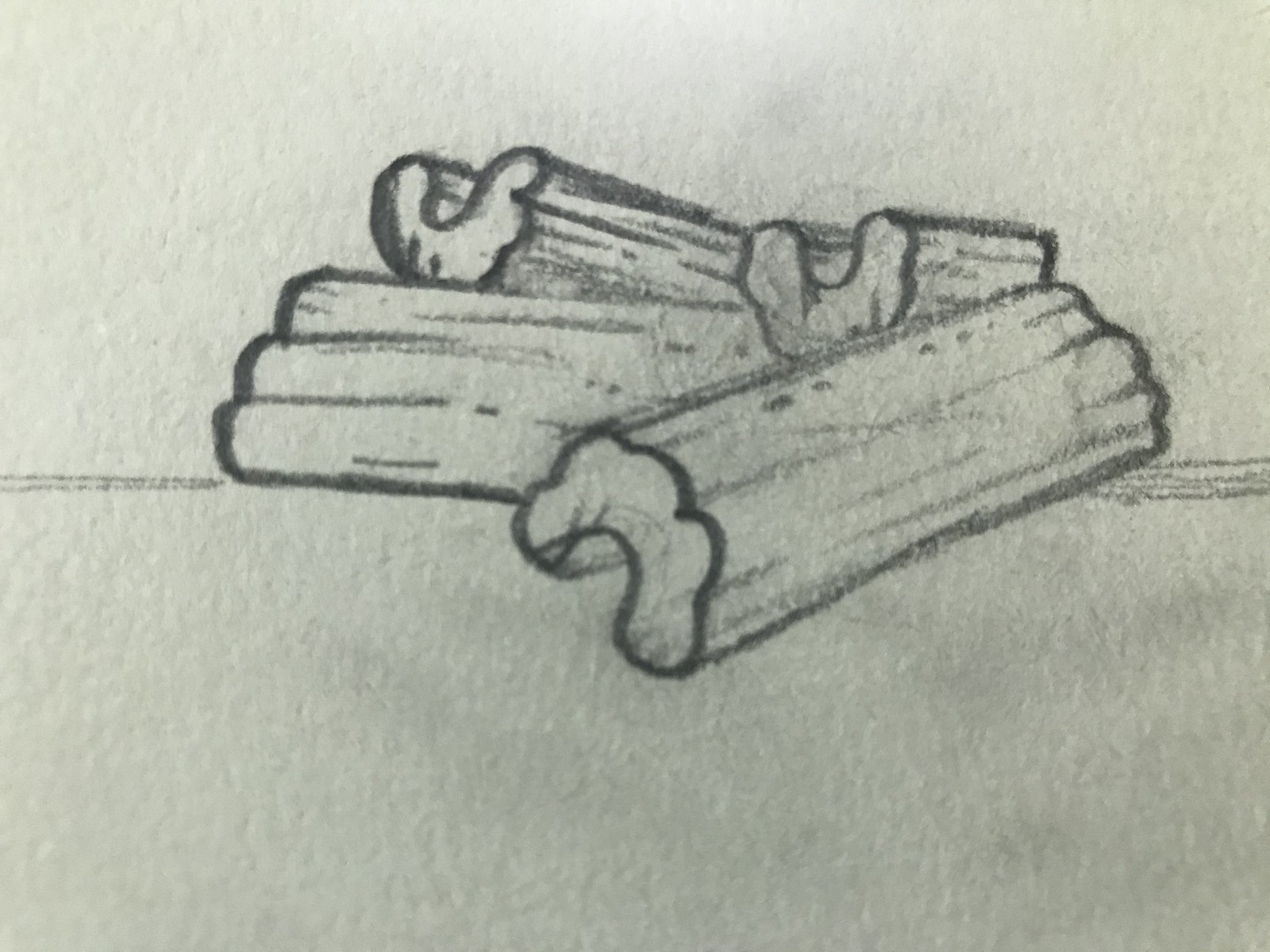This is a detailed grayscale pencil sketch on white paper, featuring four chopped pieces of celery on a surface. The drawing uses various pencil strokes to create shading and texture, with a distinct black line running horizontally across the middle of the paper, indicating the surface. On the left side of the line, the artist has included a few squiggles for added texture, while the right side has more pronounced and smudgy black pencil marks, possibly from the artist's hand.

At the center of the composition, the four celery stalks are drawn from different angles, each showcasing the hollow centers typical of celery. The pieces vary in size, with the longest extending from the right edge of the paper back towards the middle, overlapping one shorter piece. Each piece has detailed striations and shading, capturing the scalloped edges and hollow sections characteristic of celery. The sketch effectively uses large pencil strokes to convey the form and texture of the chopped vegetable.